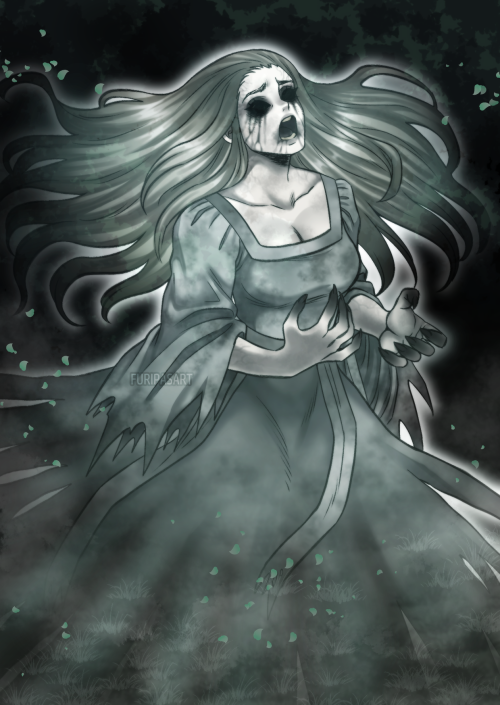The image depicts a haunting digital painting with a dark, eerie atmosphere. A weeping woman with hollow, blackened eyes, and light gray hair flowing out to her waist is the central focus. Her pale gray skin contrasts starkly with the pitch-black background, tinged with a green hue throughout the composition. Tears and trails of blood stream from her gouged-out eyes, adding to her terrifying appearance. The woman's mouth is open, as if she is screaming, while black streaks run down her face and from her mouth.

She is dressed in a billowing, tattered green dress that has a revealing neckline showing part of her cleavage. Her long, sharp fingers extend like claws, highlighted by green shadows at the tips. The dress flows in all directions, obscuring her feet, and features a jagged-edged string falling from her waist. The entire painting is speckled with light green spots and faint traces of white grass-like patterns, contributing to the surreal and frightening ambiance. In the center, there is a watermark that reads "Fury Pass Art."